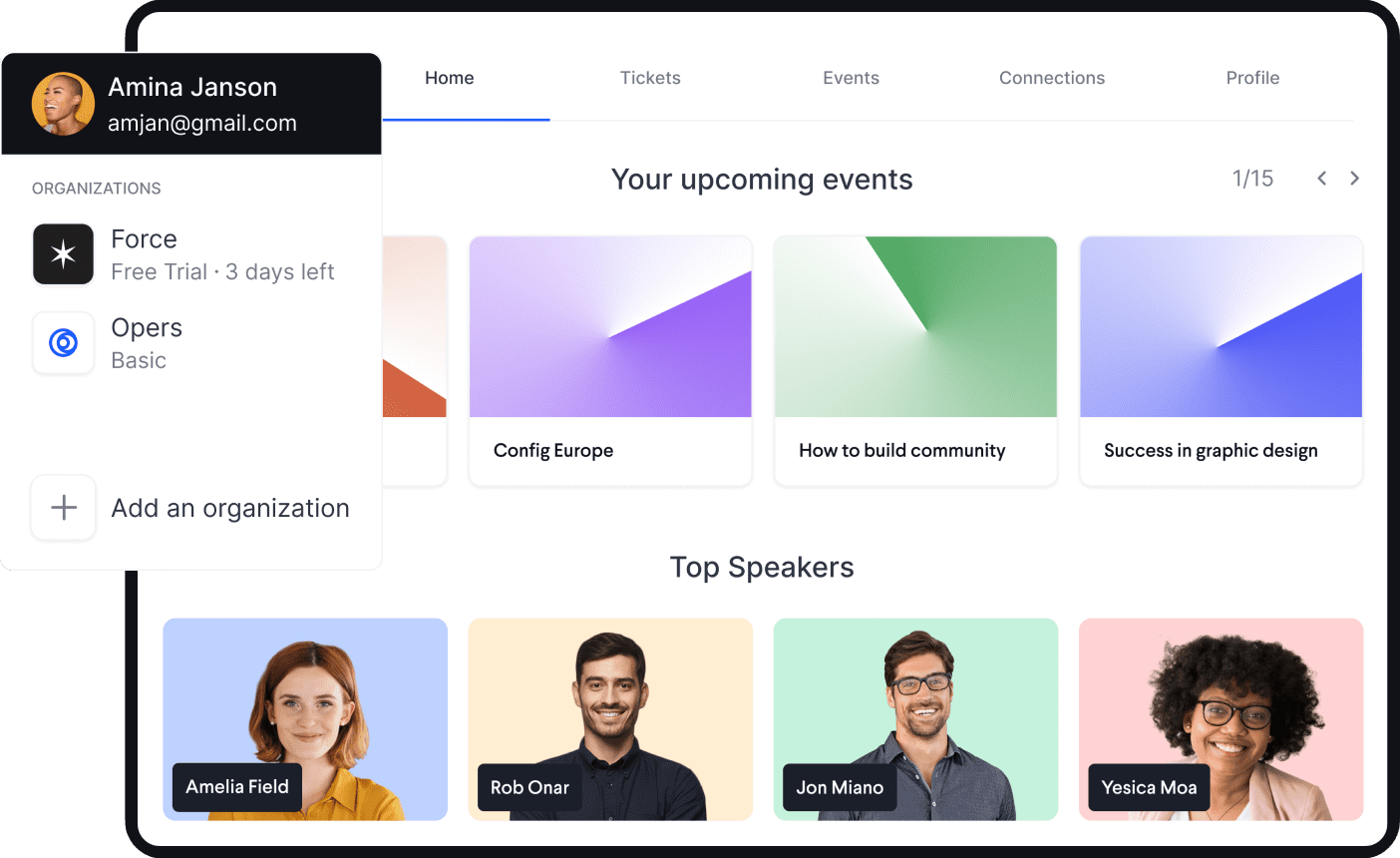The image depicts a web interface with a distinct layout and various elements. At the top, there's a black border surrounding a rectangle with a white background. Within this rectangle, the top part is black and underlined in blue with the text "Home." Next to it in gray, it reads "Tickets," "Events," "Connections," and "Profile."

On the left-hand side, a white pop-up partially obscures the content behind it. This pop-up features a user's profile picture, a woman with no hair who is smiling. Below the image, it states in white text "Amena Jameson" and underneath in black text "amjan@gmail.com." Following that, it shows "Organization: 4 Three Trout," with "3 days left" highlighted. The user is on the "Oprah's Basic" plan. There’s an option with a plus sign that says "Add an Organization."

Below this profile section, there are details about "Upcoming Events." Each event is presented in equally sized white rectangles. The first event's rectangle has a purple accent and reads "Configure a pot of build community success" focused on graphic design. The second rectangle has a green accent, and the third has a blue accent.

At the bottom, there is a section titled "Top Speakers," featuring four rectangles. The first rectangle is blue with a lady named “Amelia” written in white. The second rectangle has a yellow background with a man named “Robin R.” The third rectangle has a green background featuring a man with glasses named “John Me.” The final rectangle has a pink background with a lady wearing black glasses named “Jessica M.”